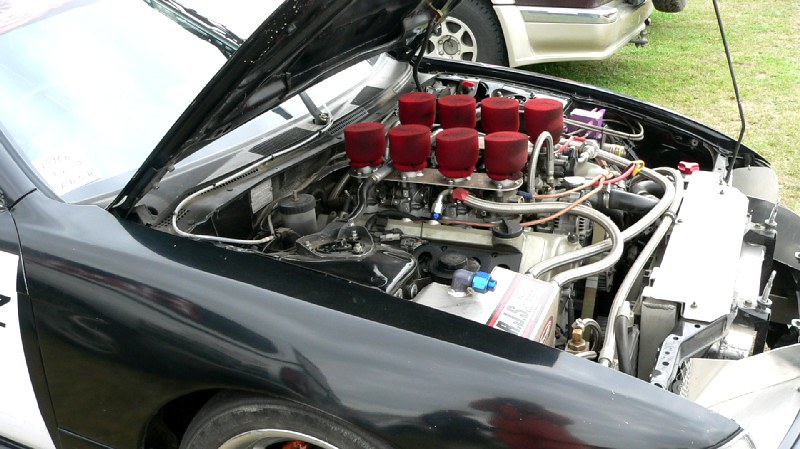This horizontal rectangular photograph, likely taken at an outdoor car show on a grassy lawn, prominently features a highly modified, black eight-cylinder muscle car with its hood raised. The car, which may have a dark green tint, showcases an extraordinary high-performance engine with evident modifications that include a distinctive fuel system and the absence of typical valve covers. The engine is adorned with eight individual red air filters arranged in two rows of four along a sleek stainless steel mounting bezel. The overall engine setup is striking, with abundant braided steel hoses snaking around top-of-the-line parts, indicating meticulous customization that enriches the fuel mixture for enhanced performance.

Notably, a vertical metal pole, partially cut off at the top edge of the photograph, supports the open hood, revealing a glimpse of the car’s front right fender and a partial view of a white sign or panel with a "Z" on the front passenger door. The image includes an additional backdrop of another light-colored car with visible tires, reinforcing the setting as a bustling car show with various vehicles displayed on the grass. The clean and gleaming engine, combined with the dark body and unique alterations, underscores the vehicle's distinguished presence among other exhibited cars.